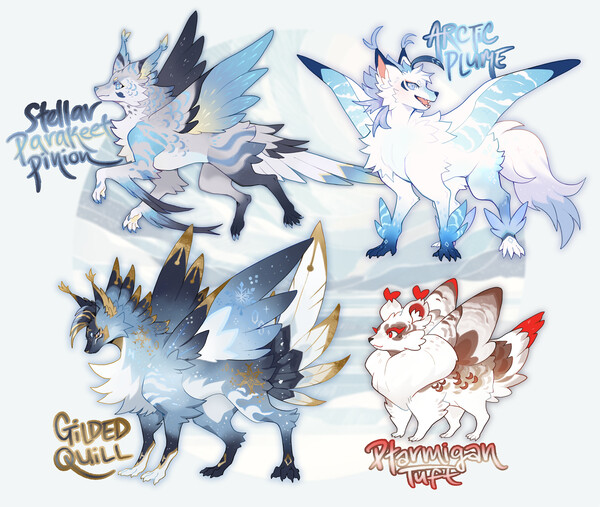The artwork features an intricate drawing of four unique, fox-like winged creatures, each accompanied by their respective names. 

Starting from the top left, the first creature, named "Stellar Parakeet Pinyon," is predominantly white, blue, and black. It bears fairy-like wings with one in black and one in blue, blue eyes, a blue nose, and has distinctively colored paws—white at the front and black at the back.

To the top right, "Arctic Plume" is a blend of very light blue and white. This creature features two blue paws, two white paws, a white bushy tail, and a wing-like structure blending white and blue tones.

On the bottom left, "Gilded Quill" presents a captivating mix of black, gold, and white along with intricate designs at the tips of its feathers or fur. It has two white paws at the front and two black paws at the back, denotatively marked in detail.

Finally, in the bottom right, "Ptarmigan Tuft" stands out with its smaller size and a color palette of white and brown with red accents at the tips. It has almost heart-shaped ears at the top, adding to its unique charm.

Each creature is depicted with an ethereal, mystical quality, reflecting a shared essence of pale blues, grays, and whites, except for "Ptarmigan Tuft," which adds a warm contrast with red and brown highlights.